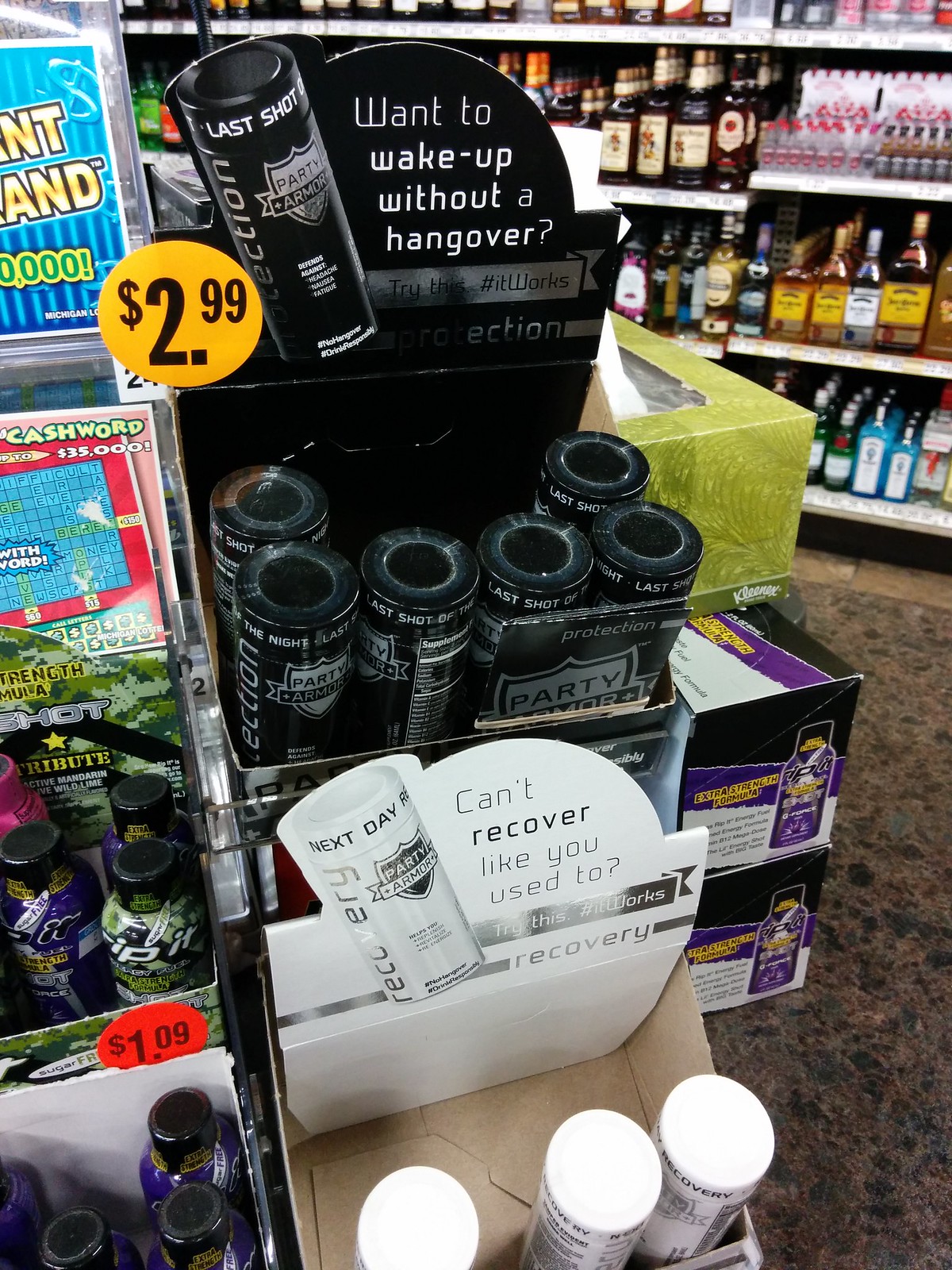The image depicts a display inside a liquor store showcasing a variety of products aimed at preventing and recovering from hangovers. The central focus of the display features prominently a black and white label that reads, "Want to wake up without a hangover?" This label is part of an advertisement for "Party Armor," a product designed to defend against headaches, nausea, and fatigue. The Party Armor cans are priced at $2.99, indicated by a yellow sticker. Beneath these, another section of the display promotes a recovery variant of the product, accompanied by smaller bottles that resemble energy shots. Alongside these are additional small energy drinks and variably colored scratch-off lottery tickets.

In the background, a variety of alcohol bottles are visible, including brands such as Fireball, Bombay, and Sailor Jerry, signifying the availability of whiskey, gin, and rum. The floor is carpeted, which is unusual for a liquor store setting. Off to the left of the display, there is another advertisement featuring blue and gold scratch-off tickets with a prominent "$35,000 Cashword" ticket. Nearby, smaller bottles of energy shots are tagged with a price of $1.09 and situated on display alongside the "Party Armor" product line.

Overall, the image captures a comprehensive view of various products aimed at enhancing consumer experiences related to alcohol consumption, from energy boosters to hangover prevention and recovery solutions, set against a backdrop of well-stocked liquor shelves.